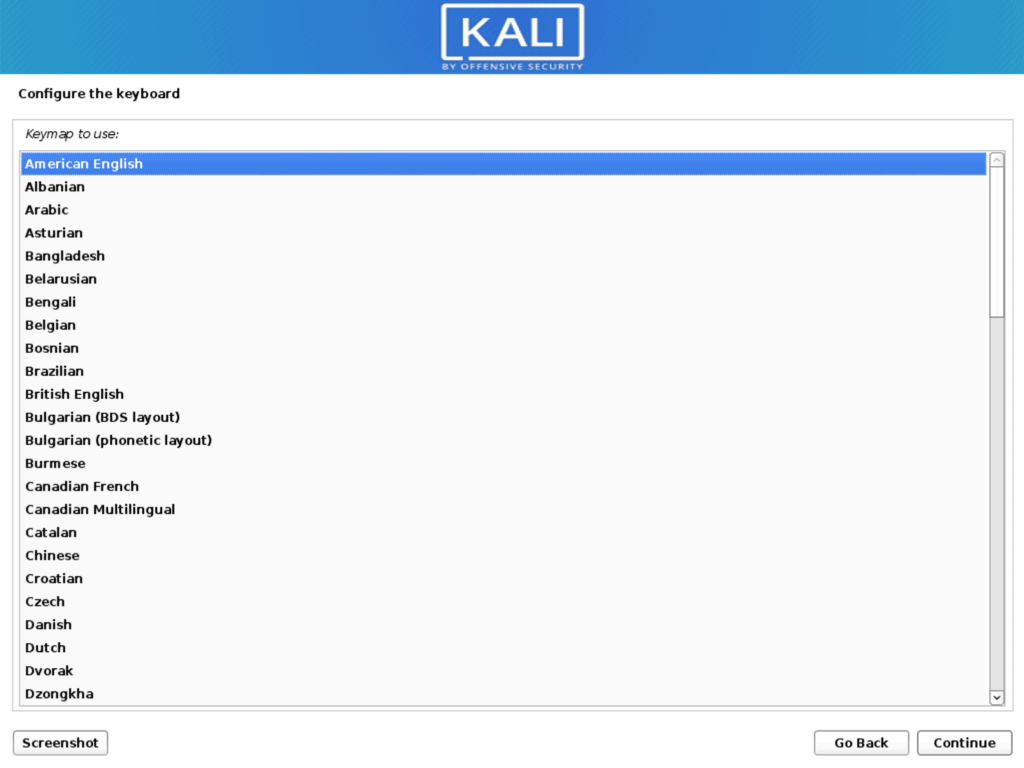Screenshot of Kali Linux by Offensive Security displaying the keyboard configuration setup screen. The header, in white font, reads "Kali by Offensive Security" and is prominently located at the center-top of the interface. The background features a gradient transitioning from light blue to dark blue and back to light blue, providing a visually pleasing contrast. Below the header, bold black text clearly states "Configure the keyboard." 

Centered beneath this title is a rectangular section containing a list of available keymaps, with "American English" highlighted in blue to indicate its selection. The extensive list of languages includes:
- Albanian
- Arabic
- Asturian
- Bangladesh
- Belarusian
- Bengali
- Belgian
- Bosnian
- Brazilian
- British English
- Bulgarian (BDS layout)
- Bulgarian (phonetic layout)
- Burmese
- Canadian French
- Canadian Multilingual
- Catalan
- Chinese
- Croatian
- Czech
- Danish
- Dutch
- Dvorak
- Dzongkha

At the bottom of the screen are three buttons, labeled "Screenshot," "Go Back," and "Continue," providing navigational options for the user.